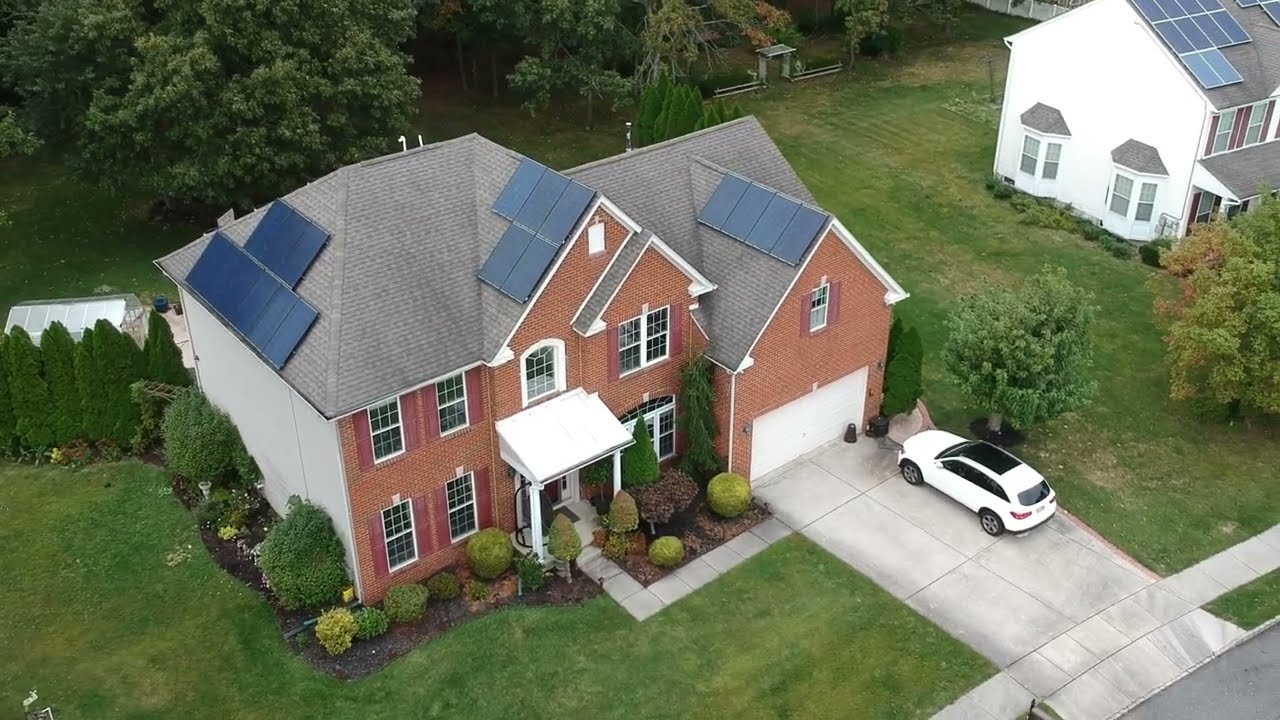This clear and bright daytime drone photograph captures an overhead view of a large, two-story brick home situated in a lush, residential suburban area. The main house, prominently featured in the center of the image, is constructed from brown bricks and features a gray roof adorned with several solar panels. The roof, which diverges in multiple directions, is lined with approximately 12 solar panels, all uniformly directed to the left. The house has a two-car garage with white doors, and a white SUV is parked in the driveway. The yard is well-maintained, featuring green grass, several bushes, and large trees both surrounding and behind the home.

The image also partially shows another home positioned in the top right corner. This secondary house is white with a gray roof that also supports solar panels and features two bay windows. Its front and back yards are also verdant with green grass. Notably, the setting of the photograph is free of people and text, enhancing the natural, serene realism of the suburban environment depicted.